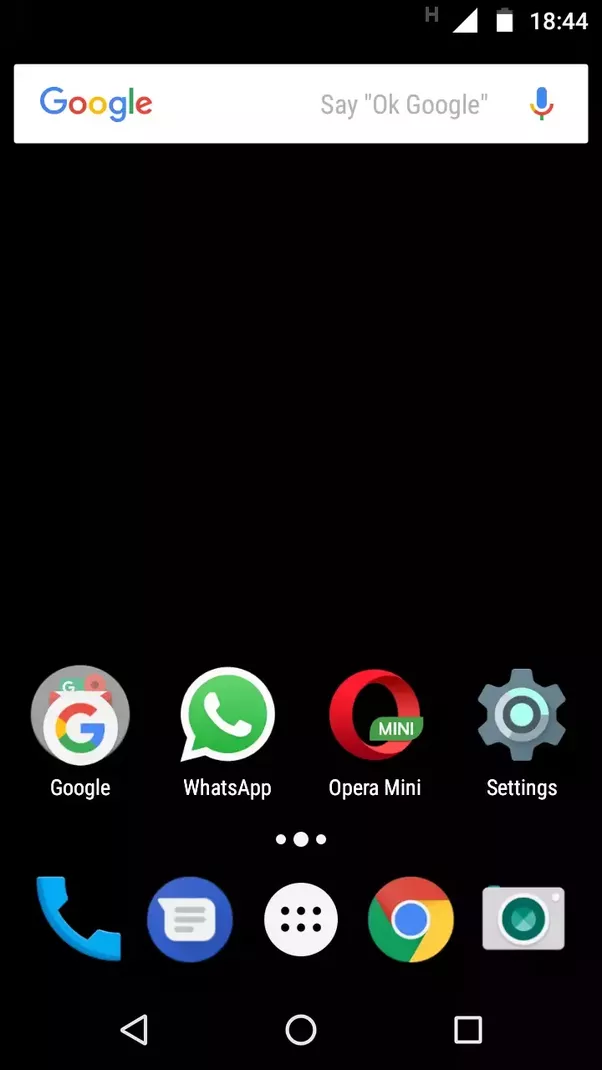Screenshot of an Android Phone Home Screen:

The image displays a screenshot of an Android phone's home screen. At the very top right, several status icons are visible: a data connectivity icon, a battery percentage indicator, and the current time, which is 18:44 (6:44 PM). Below the status bar is a Google search bar. The wallpaper in the background is solid black, enhancing the visibility of the icons and apps. The home screen features a row of app icons including Google, WhatsApp, Opera Mini, Settings, Phone, Messages, an App Library, Google Chrome, and Camera.